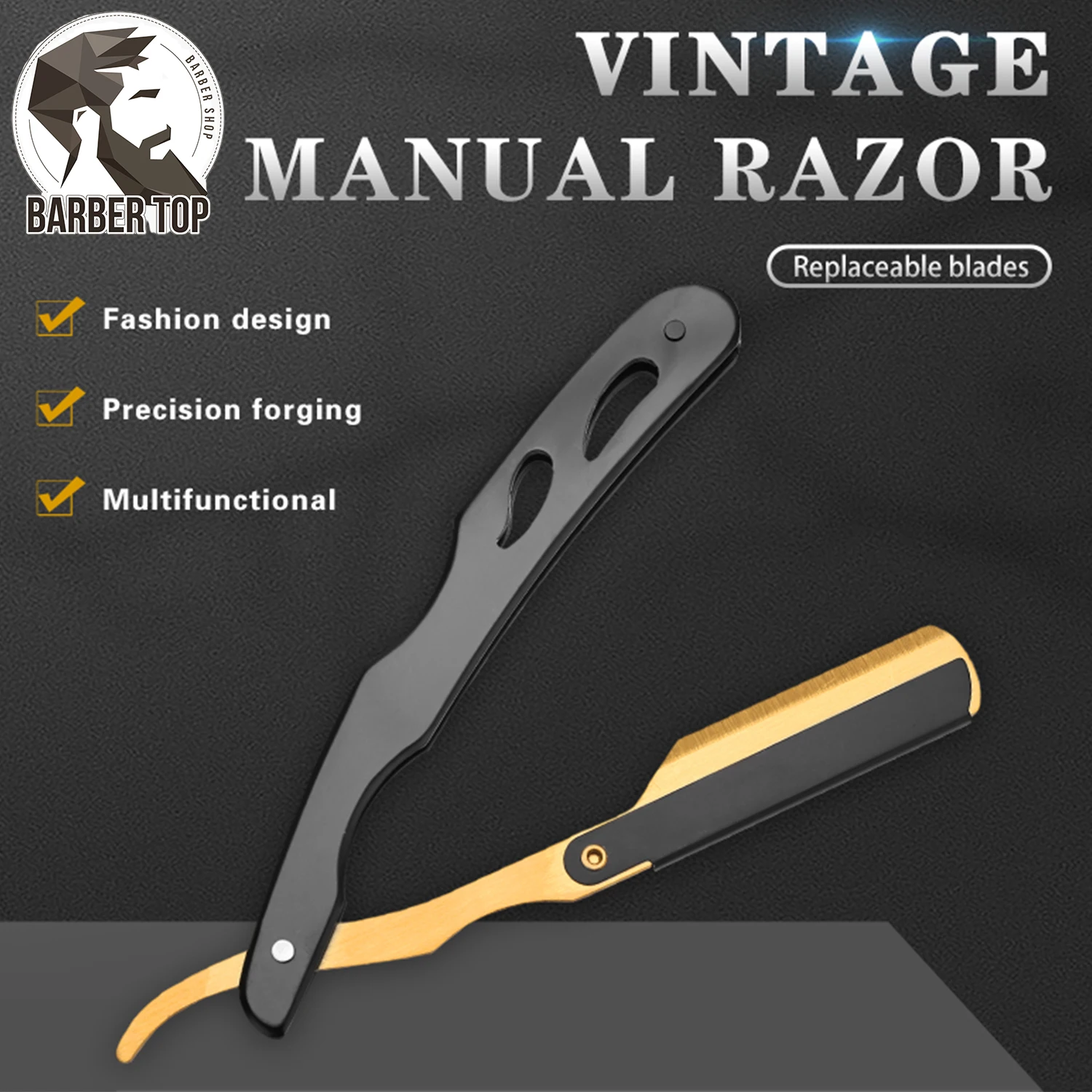The advertisement features a sleek drawing of a vintage manual razor with a replaceable blade, set against a black background. This stylish illustration showcases the razor with a black handle and a contrasting gold blade cover. In the top right corner, bold block letters read "Vintage Manual Razor," with "Replaceable Blades" written just beneath.

On the top left, a geometric profile of a bearded man with brown hair faces to the right. Underneath this image, the text reads "Barber Top" inside a white circle, with the surrounding text saying "Barber Shop." To the left of the razor, a checklist itemizes the product’s key features: Fashion Design, Precision Forging, and Multifunctional, each accompanied by a golden checkmark. Additionally, a faint blue laser-like line accentuates the 'A' in "Vintage," adding a modern touch to the classic design.

Overall, the advertisement combines elements of elegance and practicality, appealing to those who appreciate timeless grooming tools with modern enhancements.